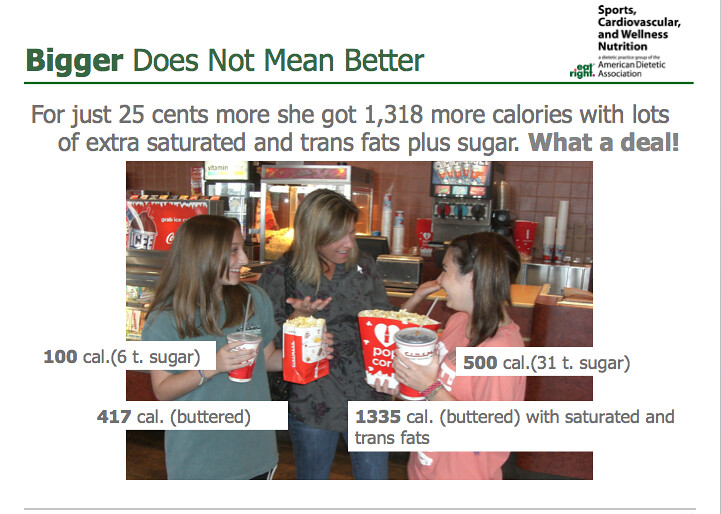The image is an informative infographic presented by the Sports, Cardiovascular, and Wellness Nutrition division of the American Dietetic Association, as indicated by the logo in the top right corner. It features a color photograph of three white females, presumably a mother with her two daughters, in what appears to be a movie theater concession area. The mother, positioned centrally and wearing a gray shirt with jeans, looks inquisitively at her daughter on the right, who has a larger popcorn bucket and soda. This daughter, who has brown hair in a side ponytail and is wearing a pink shirt, is compared to her sister, who has brown hair, a greenish-blue shirt, and holds a smaller popcorn and soda.

The text overlaying the image amplifies the message of portion control and unhealthy food choices. Across the top, in green text, the infographic declares, "Bigger does not mean better." A horizontal green line follows, under which smaller gray text warns, "For just 25 cents more she got 1,318 more calories with lots of extra saturated and trans fats plus sugar. What a deal!" Additional labels in white rectangles detail the caloric and sugar content of the snacks: the smaller soda containing 100 calories and 6 teaspoons of sugar, and the smaller buttered popcorn with 417 calories. In comparison, the larger soda has 500 calories and 31 teaspoons of sugar, and the larger buttered popcorn contains 1,335 calories with saturated and trans fats. This infographic aims to raise awareness about the nutritional impact of supersizing food and encourages consumers to make healthier choices at concession stands.